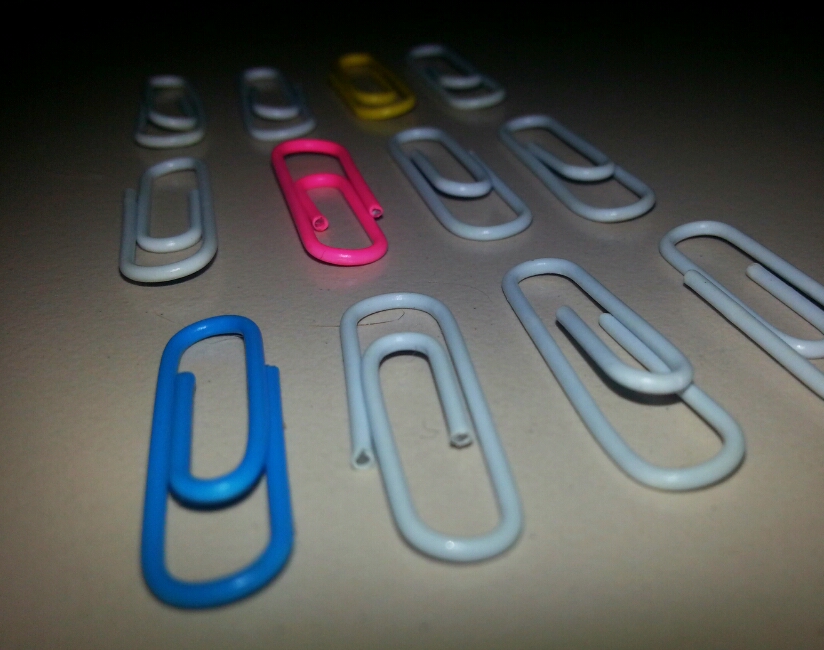This is a close-up photograph of 12 paperclips arranged neatly on a light-colored surface, taken from a low angle. The paperclips are organized in three rows of four, oriented vertically. The top row features two gray paperclips, followed by a yellow one, and another gray paperclip. In the second row, there's one gray paperclip, a pink one, and two more gray paperclips. The bottom row begins with a medium blue paperclip, followed by three gray paperclips. All the paperclips appear to be of the same brand, coated in various colored plastic. Dark shadows frame the edges and corners of the photo, with the blue paperclip in the bottom row clipping off the image's edge.